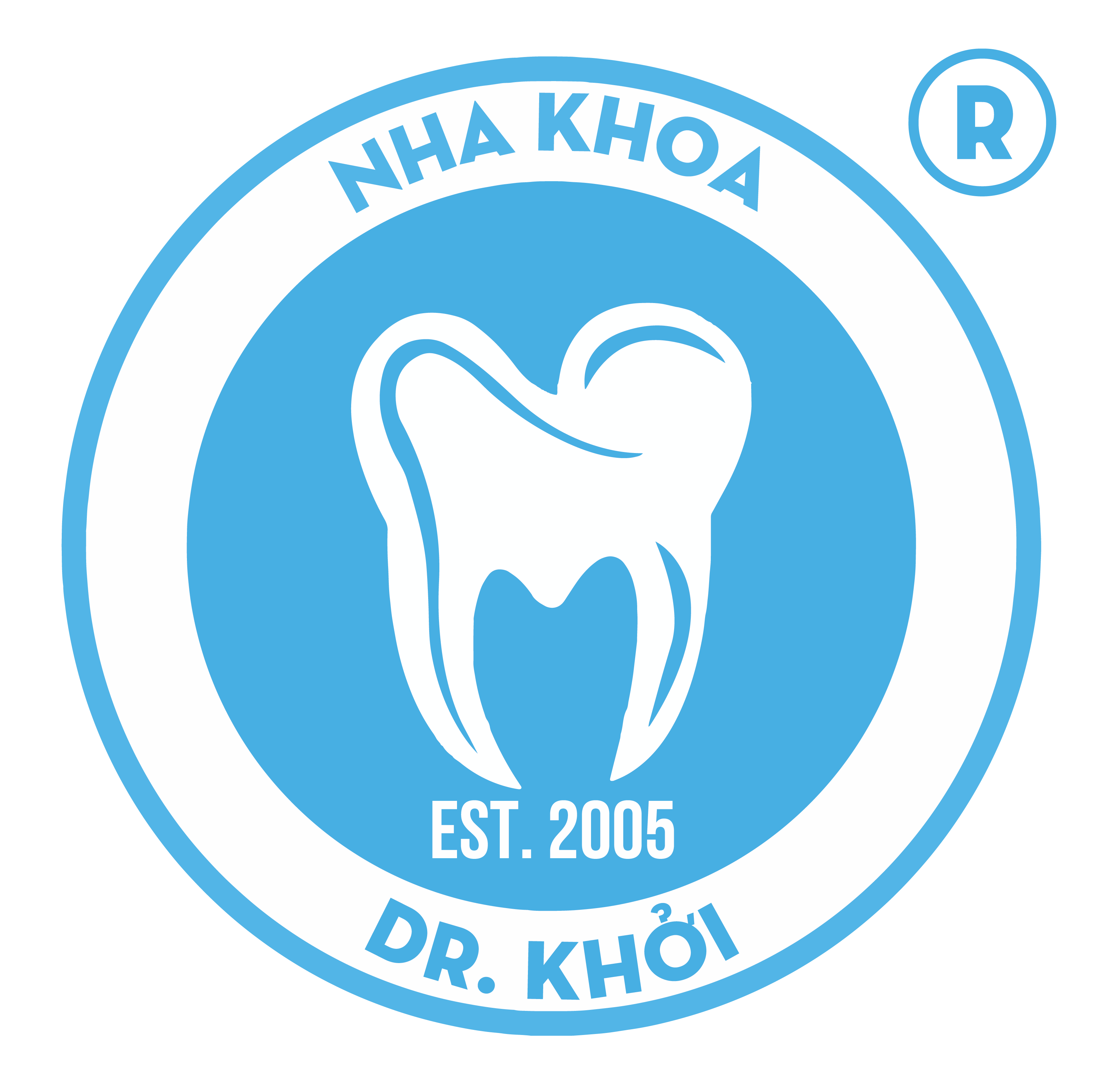The image is a detailed logo predominantly featuring shades of blue and white. The central element is a large representation of a white tooth set against a light blue background, emphasizing its importance. Below the tooth, in white text, it reads "EST.2005," indicating the establishment year of the practice.

This tooth graphic is encircled by a series of rings: immediately around it is a white ring, followed by a broader light blue ring which serves as the outermost border of the main design. Within the white ring, there is blue text at the top that bears the name "NHA KHOA," potentially indicating the dental nature of the practice, likely in Vietnamese. At the bottom within the same white ring, it says "Dr. KHOI," with the "O" accented, identifying the proprietor.

In addition to this primary circular design, there is a smaller blue ring located in the upper right portion of the image. Inside this ring is the letter "R," resembling a registered trademark symbol, adding a formal touch to the logo. This thoughtfully composed logo appears to be for a dental practice established in 2005, prominently and cleanly presenting its key details amidst the simplicity and professionalism of its color scheme and layout.